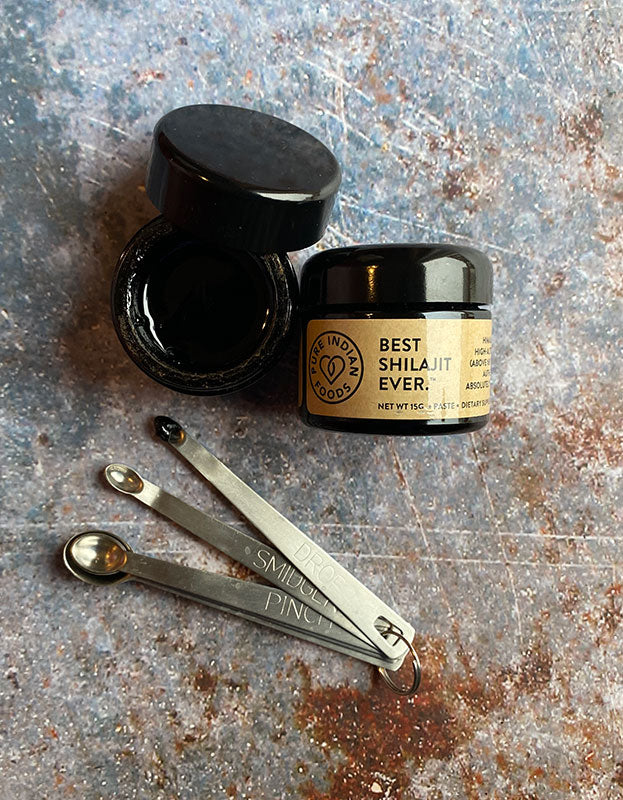This product photograph features an overhead shot of two small black containers prominently positioned on a rugged, scratched stone countertop, likely granite. The container on the left lays on its side, displaying a detailed brown label that reads "Best Shilajit Ever" and "Pure Indian Foods." Adjacent to it, another identical container stands upright with its lid removed, revealing a dark, thick liquid inside. Scattered below the containers are intricately labeled measuring spoons reading "Pinch," "Smidgen," and "Drop," indicating the high potency of the product.